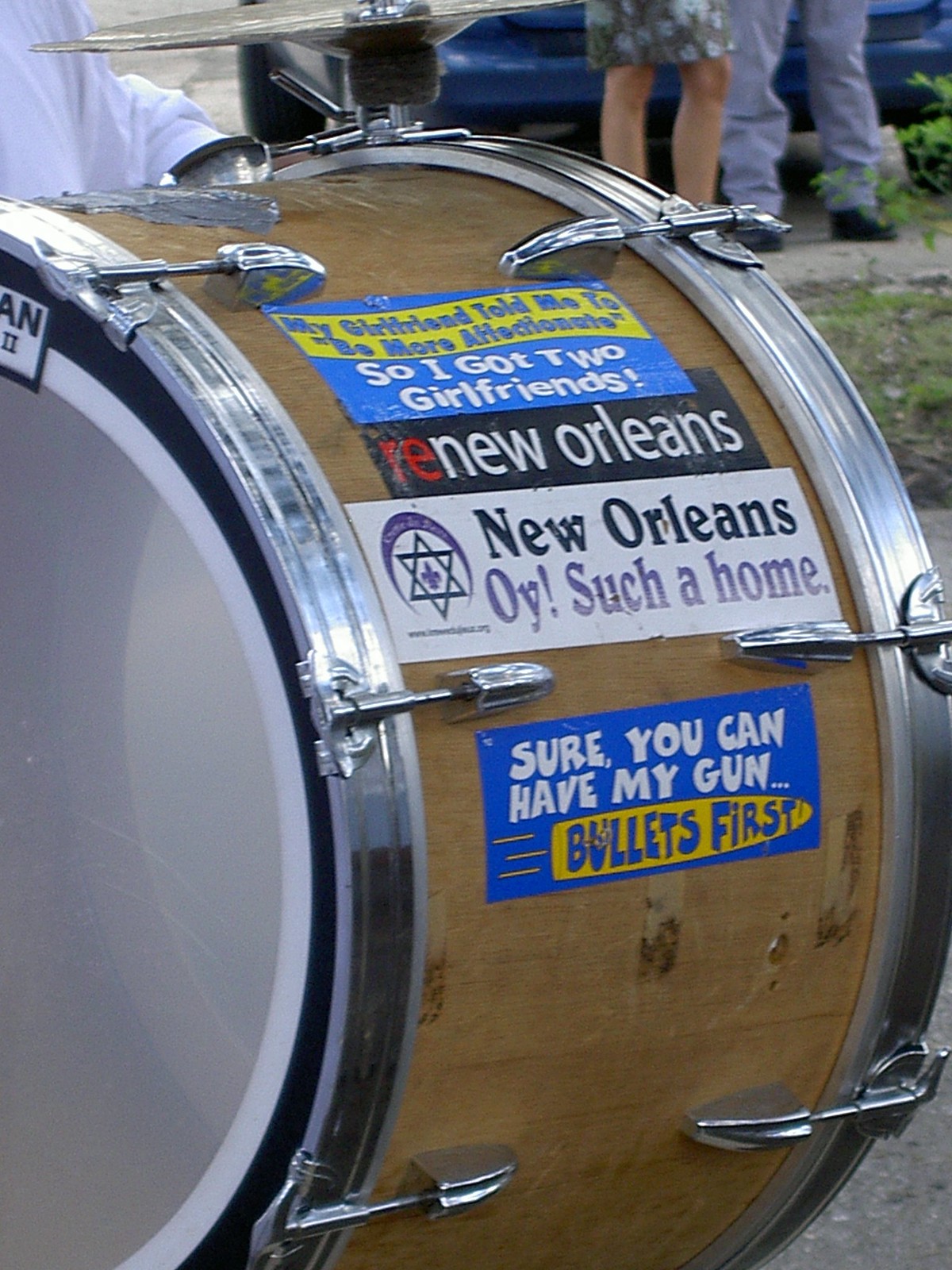The image features a close-up view of a worn, tan-colored bass drum, likely belonging to a marching band, set in a grassy area. The drum appears somewhat old with duct tape sealing it at the top, and it has a bare wooden finish with no central design or paint. Several vivid stickers are prominently displayed on the front. From top to bottom, there is a blue sticker reading, “My girlfriend told me to be more affectionate, so I got two girlfriends.” Beneath it, a black sticker says, “Renew Orleans.” Following that is a white sticker featuring the text, “New Orleans, oy, such a home.” Further down, another blue sticker reads, “Sure, you can have my gun,” with the additional caption “bullets first” nearby. The image's background reveals partial views of people, including legs clad in jeans and black shoes, and another person wearing a green skirt with blue flowers, as well as some scattered leaves. The overall quality of the image appears low-resolution, suggesting it might be a screenshot from a video, capturing movement and activity around the drum.